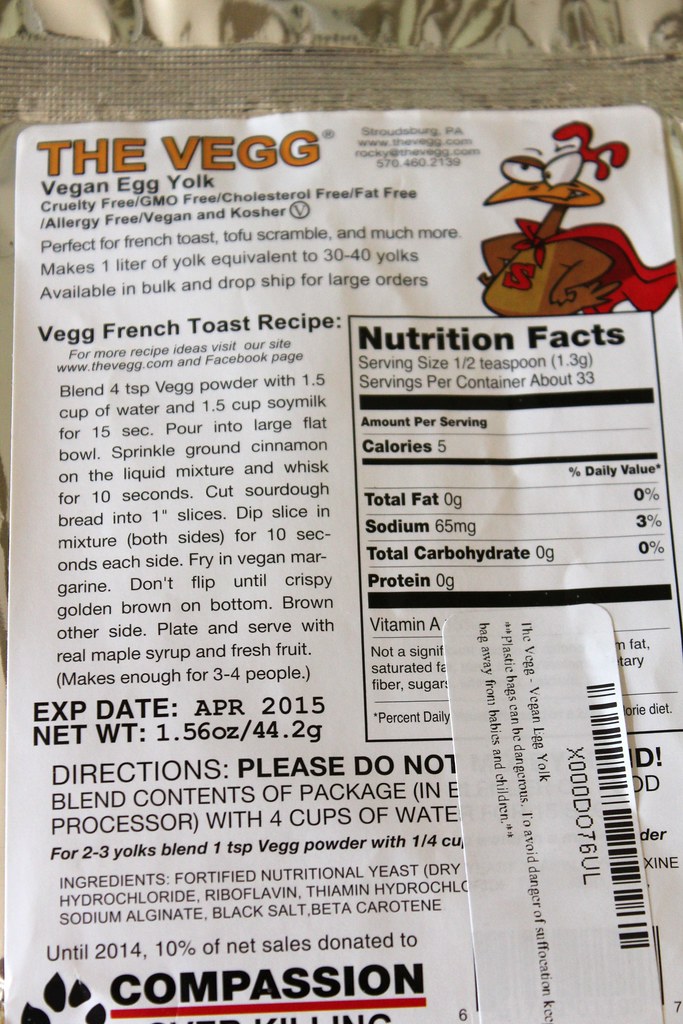This image displays the back label of a food package with various sections providing detailed information. At the top, there is a white, rounded-edge triangular label featuring the word "VEG" in bold yellow lettering. Below this, a description in black font elaborates on the vegan egg yolk contained within the package. Adjacent to the description, a recipe for vegan French toast is presented in a clear and user-friendly format. At the bottom of the label, essential details such as expiration dates, usage directions, and additional information are provided. On the right-hand side, a comprehensive nutrition label outlines the product's dietary content. Additionally, a whimsical cartoon turkey, adorned in a red cape with an 'S' emblem on its chest, adds a playful touch to the design. Another sticker label can be seen in the bottom-right corner of the image.